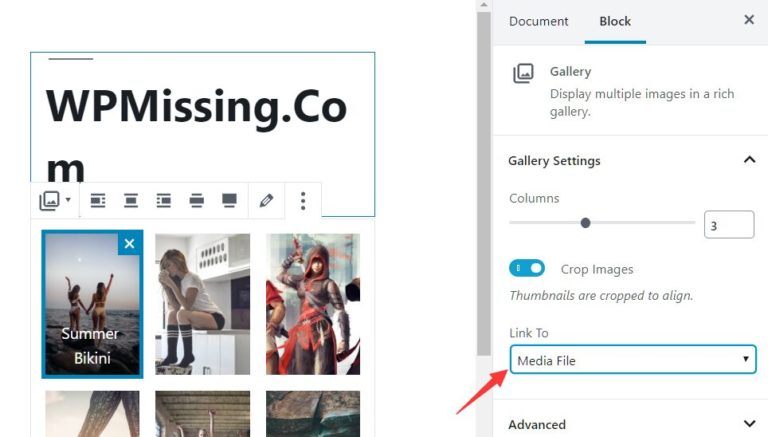**Detailed Caption:**

The image is divided into two distinct sections on a white background. The left section features a large rectangular outline with a thin Tiffany blue line. Prominently displayed within this section is the text "WPmissing.com." This text is creatively styled: "WPM" is in capitalized, big black letters; "missing" follows with an uppercase "M" at the beginning, and the "C-O-M" part is positioned so that the "M" is directly beneath the capital "W." Just above the "W" is a subtle gray line.

Below "WPmissing.com," there are several icons, followed by two rows of images, with the bottom row partially visible. The top row contains three distinct pictures. The first image on the top left has a Tiffany blue outline and contains a Tiffany blue box with a white "X" in the top right corner. This image is captioned "Summer Bikini" in white text and features two girls in bikinis, one reaching up with her right arm, and the other reaching up with her left arm, set against a backdrop of the ocean and a gray sky.

The middle top image depicts a girl sitting on a countertop, wearing a white t-shirt and knee socks. The background consists of white furniture, creating a clean and monochromatic appearance. The final image on the top right shows a person dressed in a warrior outfit, possibly from a video game, with gray and red clothing and a hood. This character is raising their right arm, and there is another individual to the left wearing a red shirt, set against a mixed background of pale green, gray, and orange hues.

The bottom row of images is mostly obscured, showing only the top parts, which are cream-colored, brown, and slightly green, making the subjects indiscernible.

The right section of the image is entirely text-based and includes various settings and descriptions. At the top, "document" is written in gray, with "block" in a darker gray underlined in Tiffany blue on the right side. A small "X" is located on the far right. Below, on a white background, the text "gallery" appears alongside a picture icon, with the description "display multiple images in a rich gallery" in gray below it. A medium gray scroll bar is on the left side.

Further down, the section labeled "gallery settings" is written in dark gray, followed by "columns" in light gray with a horizontal gray line beneath. Near what would represent the number three in this context, a black dot is present, and to the right of it, the number "3" appears in a box. Below, a Tiffany blue ellipse features a white circle on its right side, and beside it, the phrase "crop images" is displayed in gray. The text "thumbnails are cropped to a line" is in italics below, also in gray. 

Continuing, "link to" is written in gray, followed by a wide white rectangle outlined in Tiffany blue, containing the text "media file" with a drop-down indication. A red arrow points up towards "media file" from the bottom left, with the arrow tapering at the bottom. The final row states "advanced," accompanied by an arrowhead pointing downwards.